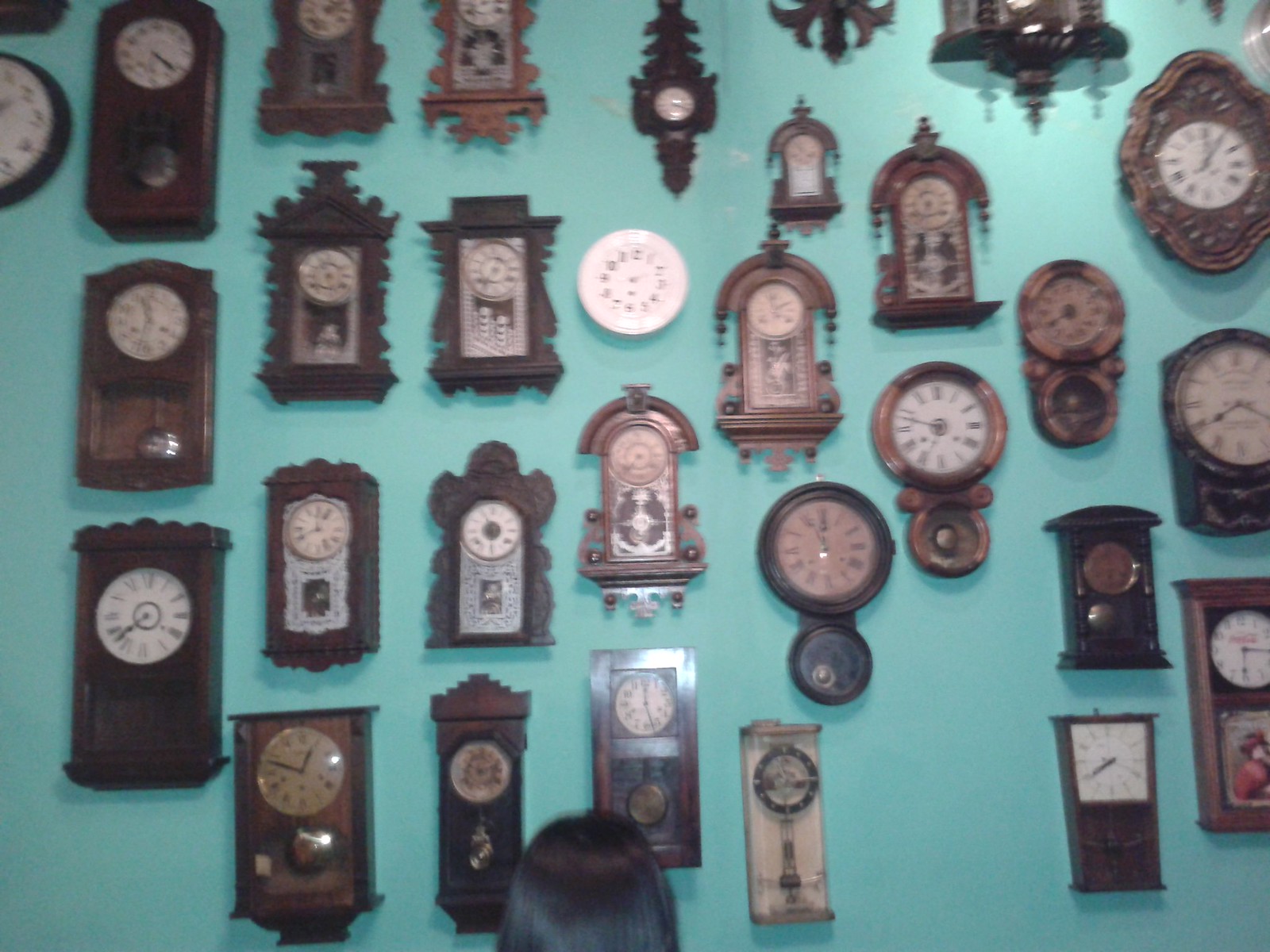The image showcases a visually striking teal or turquoise wall adorned with an eclectic collection of antique wall clocks. The arrangement features both round and rectangular clocks, most of which are made of beautifully polished wood with intricate carvings. The clocks exhibit a mix of Roman numerals and standard numbers on their analog faces, and many are modeled after miniature grandfather clocks, complete with hanging mechanisms. In the center of the display, there is a standout white round clock, surrounded by a seemingly haphazard yet artistically pleasing arrangement of various other timepieces, totaling approximately eight across and three to four down. The spacing between each clock is intentional, leaving a few inches of teal wall visible around each. The bottom of the image subtly includes the black hair of a woman, observing the captivating assortment of clocks.